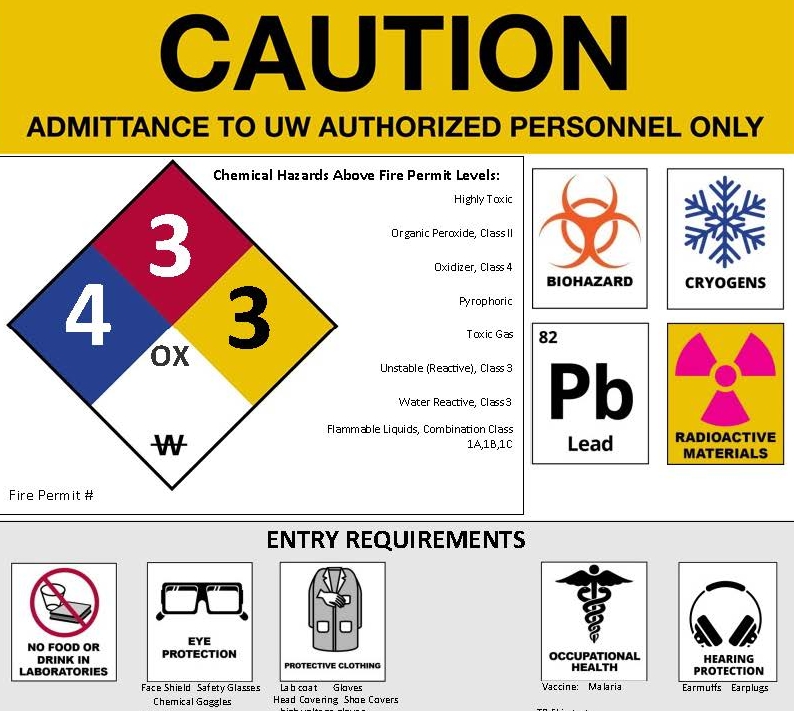The image is a comprehensive safety poster designed for a hazardous materials area, likely within a workplace or laboratory setting. Dominating the top portion, the word 'Caution' is boldly displayed in large black capital letters against an orange striped background. Directly beneath, a warning message reads, "Admittance to UW Authorized Personnel Only."

The middle section features a grid of hazard symbols. These include an orange biohazard symbol, a blue cryogen symbol represented by a snowflake, the chemical symbol for lead (Pb), and a yellow square with a hot pink radioactive materials symbol.

Adjacent to these, on the left side, the sign elaborates on additional chemical hazards like high toxicity, organic peroxide, and flammable liquids. A diamond-shaped NFPA (National Fire Protection Association) label is also present, divided into four sections: a red section with the number '3' indicating flammability, a yellow section with the number '3' signifying reactivity, a blue section with the number '4' for health hazards, and a white section labeled 'OX' for oxidative hazards with a 'W' crossed out indicating it reacts with water.

At the bottom of the poster, there’s a gray strip outlining the entry requirements: prohibiting food and drink, mandating eye protection and protective clothing, and stipulating the use of hearing protection. Notable icons include a food and drink prohibition symbol, goggles, a lab coat, a medical emblem denoting occupational health, and headphones indicating required hearing protection.